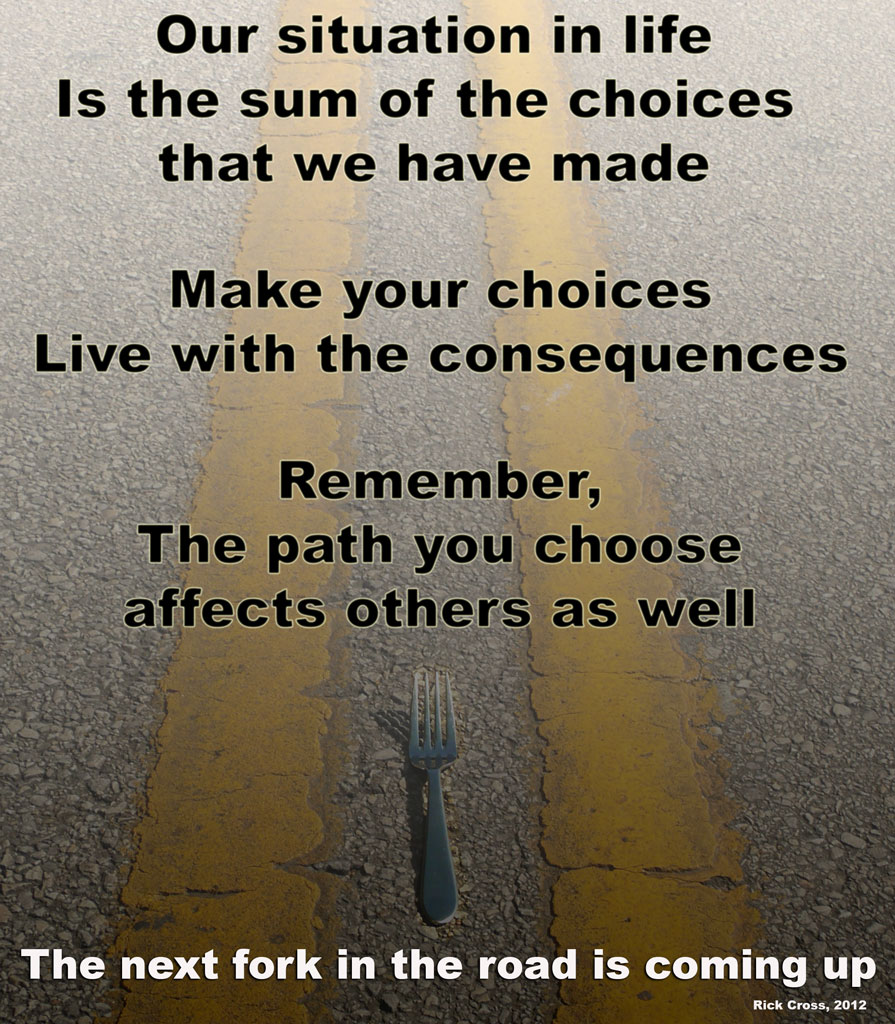The image features a weathered asphalt roadway with a pronounced center line composed of two solid yellow lines that run from the bottom to the top of the image. Between these lines, at the bottom center, lies a silver eating fork, creating a visual pun. The yellow lines exhibit signs of aging, with cracks and crumbling edges. Dominating the upper and central parts of the image is a black text overlay that reads, "Our situation in life is the sum of the choices that we have made. Make your choices, live with the consequences, remember the path you choose affects others as well." At the very bottom, in white text, it states, "The next fork in the road is coming up," with a smaller font crediting "Rick Cross 2012" in the lower right corner. The background is a stark, cracked road surface, contrasting with the clean, striking messages presented.